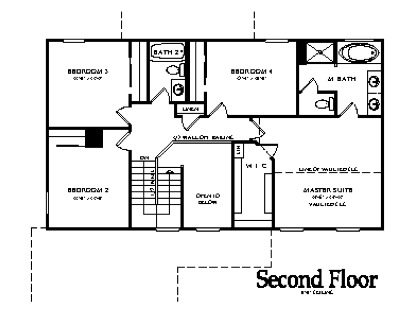This black and white blueprint depicts the second-floor layout of a house. At the bottom of the blueprint, the label "Second Floor" is clearly visible. The design showcases a spacious floor plan with four bedrooms, including one labeled as a "Master Suite." Two bathrooms are also present, with one providing en suite access to two bedrooms. A central hallway connects all the rooms, each featuring distinct entrances. The plan includes a versatile room that could serve as a living space or flex area, although its specific purpose is not indicated. Various measurements and dimensions are meticulously marked throughout the blueprint. Breaking lines at both the bottom and top of the layout suggest transitional areas or stair accesses. Overall, this highly detailed floor plan emphasizes the precise organization and thoughtful partitioning of living spaces within the house.